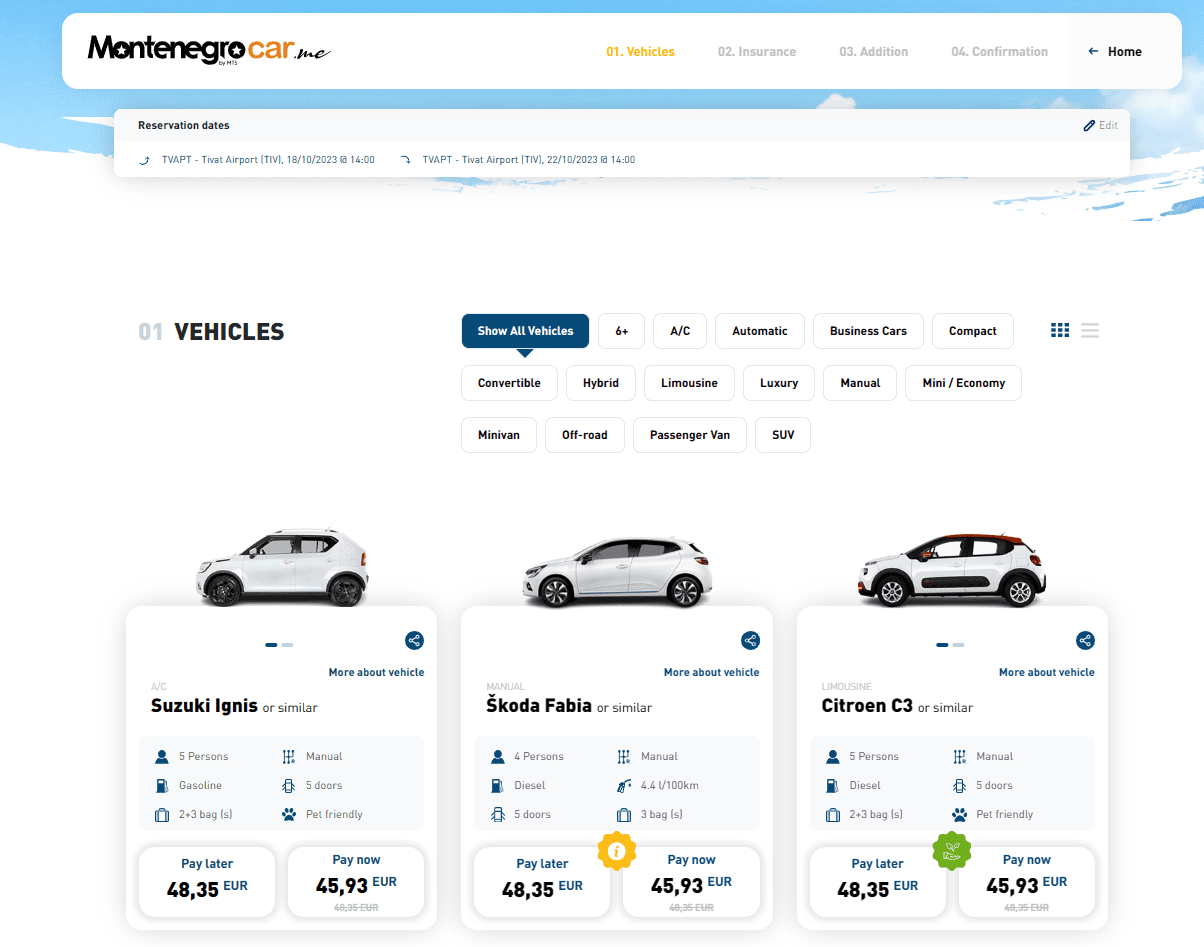The image showcases a detailed snapshot of a car rental webpage from MontenegroCar.me. The top of the webpage features a logo for MontenegroCar on the left side of a white rectangular bar, with the words "MontenegroCar.me" prominently displayed. Adjacent to the logo, "01.vehicles" is highlighted in orange, indicating the current section of the site, while the subsequent stages—"02.insurance," "03.addition," and "04.confirmation"—are faded in light gray. Further to the right, there is a navigation option labeled "home" in bold black letters accompanied by a blue left-pointing arrow.

Beneath this, a white rectangle labeled "reservation dates" shows the car rental details with the text: "going TVAPT Tevat Airport TIV 18-10-2023 at 1400" and "returning TVAPT Tevat Airport TIV 22-10-2023 at 1400," indicating a four-day rental period.

The main body of the page is headed by "vehicles" in bold black letters next to "01" in light gray. This section lists three cars available for rent, under a navigation bar with options to filter the listings. The default filter "show all vehicles" is highlighted in white with a blue background, while other options (such as "6+", "AC," "automatic," "business cars," "compact," "convertible," "hybrid," "limousine," "luxury," "manual," "mini/economy," "minivan," "off-road," "passenger van," and "SUV") are unselected and displayed in a series of tabs.

The first car displayed is a "Suzuki Ignis or similar," equipped with air conditioning (AC), five seats, gasoline engine, manual transmission, five doors, capacity for two to three bags, and is pet-friendly. Rental options are €48.35 payable later or €45.93 payable now, with the later price crossed out.

The second car is a "manual Skoda Fabia or similar," seating four persons, running on diesel, featuring five doors, and a fuel consumption of €4.41 per 100 kilometers. It also accommodates about three bags. The pay later price is €48.35 and the pay now price is €45.93, with the higher price crossed out. A distinguishing yellow sunflower-like icon with a lowercase white "i" is also present.

The third car is a "limousine Citroen C3 or similar," offering seats for five persons, diesel engine, manual transmission, five doors, capacity for two to three bags, and pet-friendly options. Additionally, it features a green hand symbol indicating eco-friendly aspects. The pay later price is €48.35, crossed out beside a pay now price of €45.93.

All cars are displayed horizontally with their front windshields on the left and backs on the right. The webpage layout is visually clear, navigating users through the rental process from vehicle selection to the final confirmation.